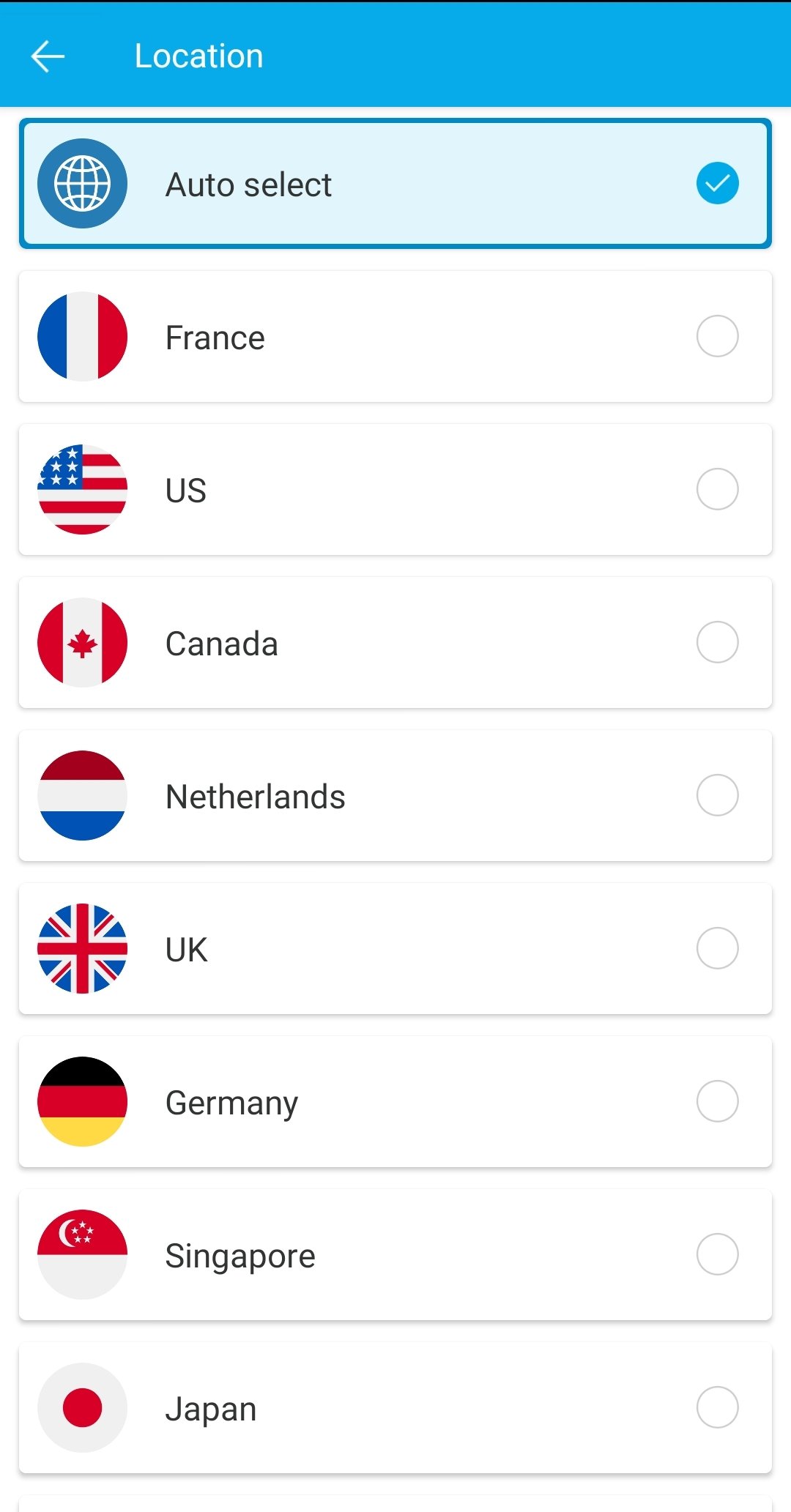The image showcases various options for selecting national flags, organized within a user interface. At the top, there is a blue bar indicating the current selection criteria. Below this selection criteria, there are multiple spheres available for auto-selection, each marked with a blue checkmark and labeled by country names along with descriptions.

1. **France:** 
    - Blue, white, and red colored circle.

2. **U.S.:**
    - Intended to be depicted as white, red, white, red stripes with the top left corner featuring a blue square (currently should be corrected as it's noted not to be red).

3. **Canada:**
    - Red, white, and red bands with a maple leaf in the center.

4. **Netherlands:**
    - Red, white, and blue arranged in horizontal stripes.

5. **U.K.:**
    - Refers to the Union Jack, likely featuring crosses of red and white over a blue field.

6. **Germany:**
    - Horizontal bands of black, red, and yellow.

7. **Singapore:**
    - Red with a white crescent moon and five white stars at the top left.

8. **Japan:**
    - A white circle with a red dot in the middle representing the Japanese flag.

Different kinds of circles are present, some of which are unchecked. At the very top, there is an overarching circle with a checkmark on it, indicating the current selection.